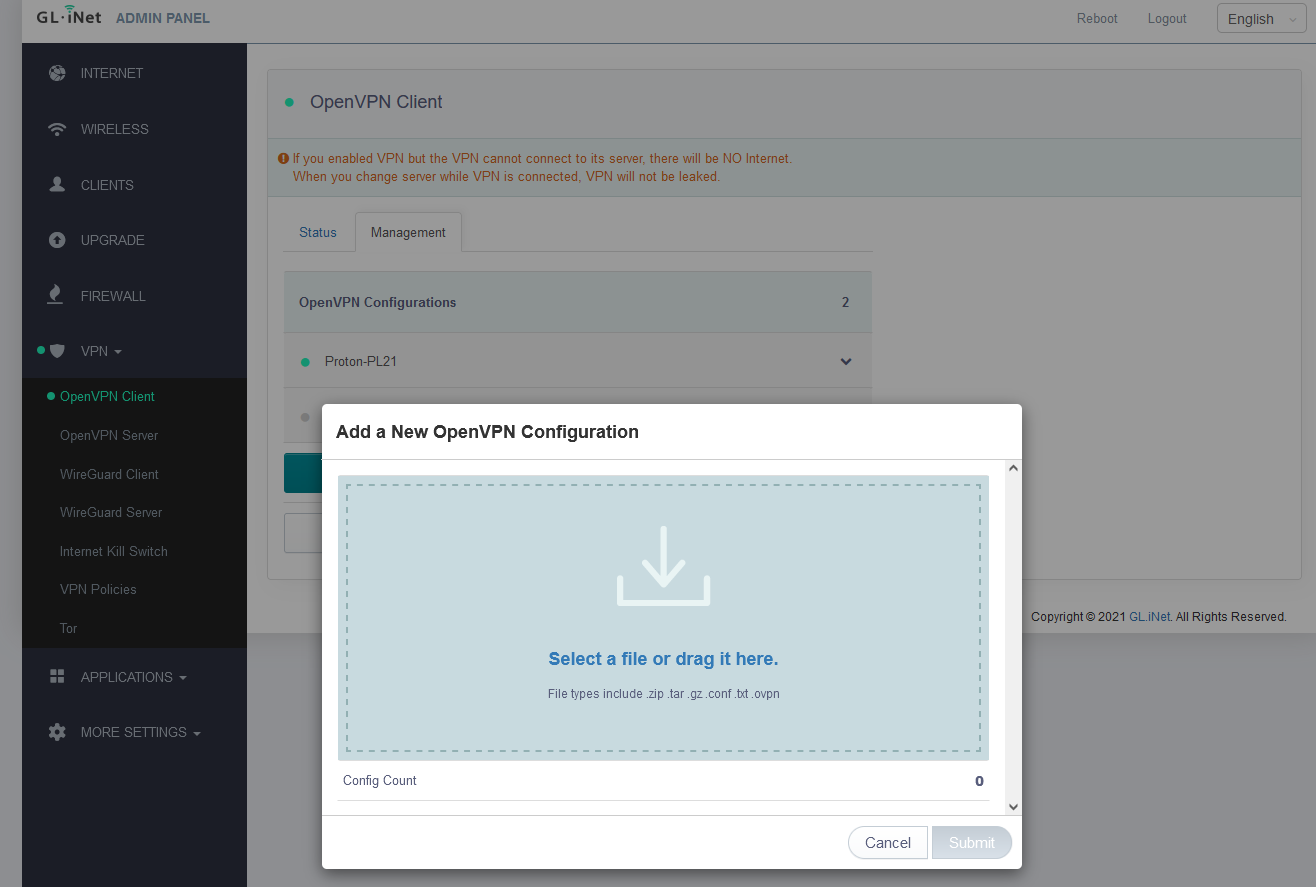This screenshot showcases an admin panel from GLINET. Positioned in the upper left corner is the GLINET logo. In the upper right corner, there are three buttons labeled Reboot, Logout, and English. The left side of the page features a vertical menu with a black background, displaying gray text and icons. Dominating the center of the screen, the main heading "Open VPN Client" is highlighted in green text, accompanied by a green circle indicator.

The majority of the screen has a white background, reiterating "Open VPN Client" with a small green dot preceding it. Below this, a red circle with an exclamation mark precedes a warning message in red text: "If you enabled VPN but the VPN cannot connect to its server, there will be no internet. When you change the server while VPN is connected, VPN will not be leaked."

At the top of this section, there are two selectable tabs titled Status and Management. Superimposed over this main window is a smaller popup window containing the instruction: "Add a new Open VPN configuration."